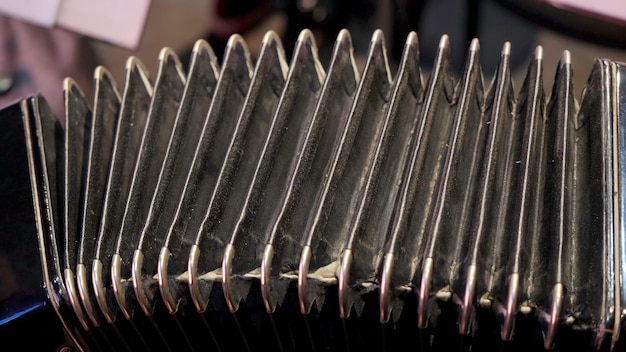This close-up photograph features the expandable bellows of an accordion, prominently stretched out and forming a convex arc across the frame. The accordion's bellows, mainly black with silver-tipped edges, dominate the image, showcasing their worn and well-used leather or fabric material. Metal corners protect the accordion's edges, which appear on the very left and right sides of the image. The frame is filled almost entirely by the accordion, with only a small, out-of-focus strip along the top hinting at an open book or sheet music on the upper left and possibly some furniture on the right. The primary colors are black, gray, and tan, and no person is visible holding the instrument. The background remains blurred and indistinct, ensuring the viewer's focus remains on the detailed, arched bellows of the accordion.